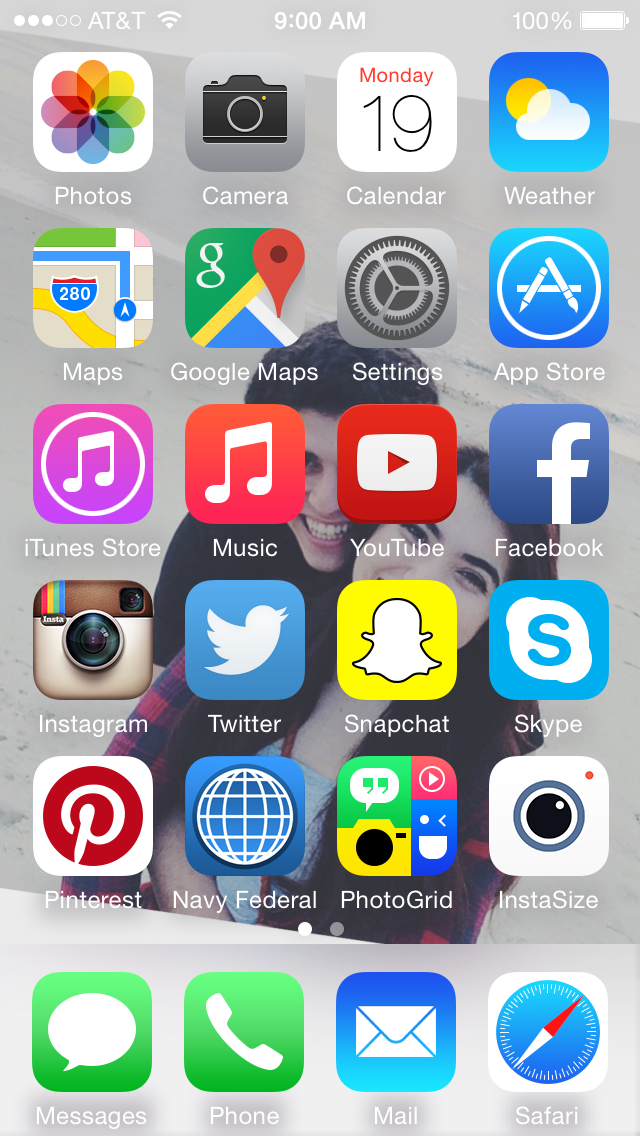This image depicts an iPhone screen showcasing various app icons. The iPhone's wallpaper features a couple, both smiling warmly. The young man, with medium-length black hair, is dressed in a black jacket or shirt and is embracing the woman from behind. The woman, with dark black eyebrows and black hair, is wearing a gray shirt layered with a red and black plaid shirt. Both appear joyous and content.

At the top of the screen, the status bar indicates the device is connected to the AT&T network with a cell signal strength of three out of five bars and full Wi-Fi signal strength. The time displayed is 9 a.m., and the battery is fully charged at 100%.

The app icons visible on the screen include:
- Photos
- Camera
- Calendar
- Weather
- Maps
- Google Maps
- Settings
- App Store
- iTunes Store
- Music
- YouTube
- Facebook
- Instagram
- Twitter
- Snapchat
- Skype
- Pinterest
- Navy Federal
- PhotoGrid
- InstaSize
- Messages
- Phone
- Mail
- Safari

Each app is neatly arranged, providing a clear and organized view of commonly used applications on the iPhone.